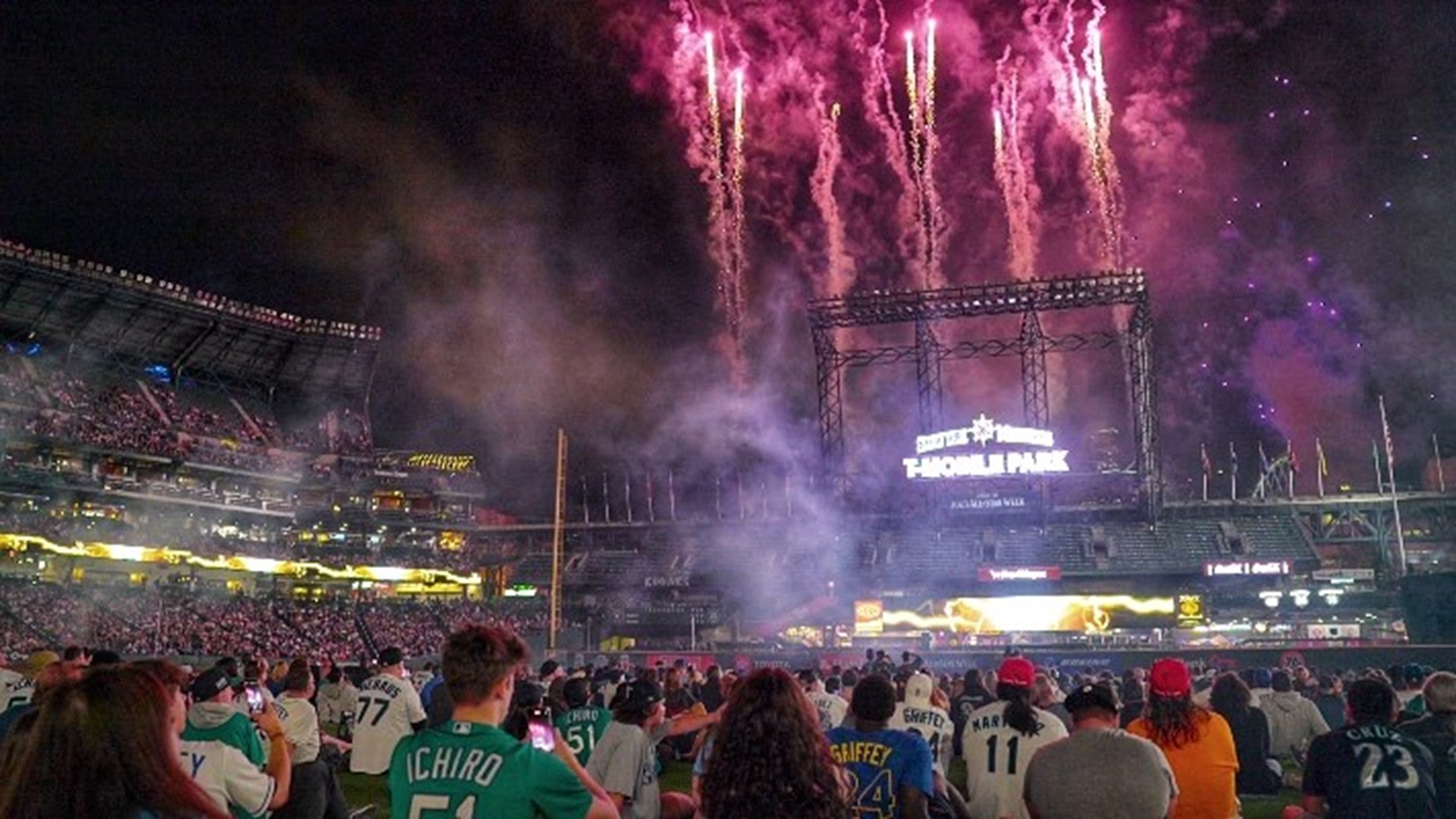This detailed photograph captures a lively nighttime event at T-Mobile Park, potentially a sporting event or concert. The image is shot in landscape orientation, showcasing a bustling stadium filled to capacity. The dark night sky looms above, contrasting vividly with the bright spectacle below. In the foreground, numerous attendees stand on the floor level, dressed in a variety of sports jerseys in colors such as green, white, orange, and blue, contributing to the vibrant mosaic of the crowd.

Dominating the center of the photograph are pyrotechnics, spraying pink and white fireworks high into the air, adding a dramatic flair to the event. The backdrop reveals a large jumbotron or stage, capturing the attention of the excited audience, many of whom have their cameras out to record the moment. The stands, cascading up the left side of the image, are packed with spectators, with the stadium's rafters and overhang visible above them, framing the enthusiastic crowd. The scene is electrified by the dazzling display, encapsulating the thrill and spectacle of the event at T-Mobile Park.